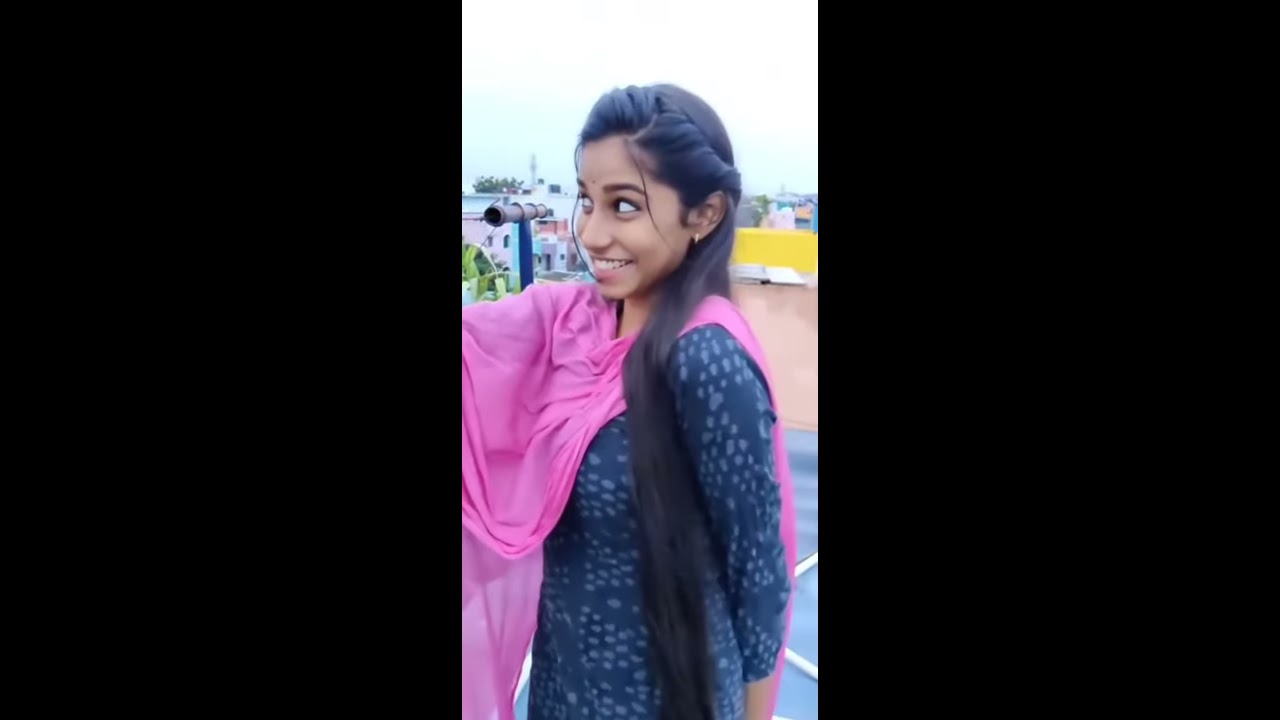The image is set in a horizontal rectangle and divided into three panels, with the left and right panels being slightly larger than the middle one. The middle panel features a young South Asian woman standing in a 45-degree profile to the left, smiling widely and looking excited. She has long, blackish-brown hair styled with slight braids at the top, cascading down below her waist, with a few loose locks framing her face. She is dressed in a blue dress adorned with lighter blue dots and wears gold earrings. Draped across her is a light bubblegum pink shawl or long, thin, sheer scarf that wraps around her body and over her back. Behind her, some buildings and a bright yellow rectangular area are visible, along with a bit of sky that appears very bright and white. The side panels on the left and right of this middle image are entirely black, framing the central image of the woman.